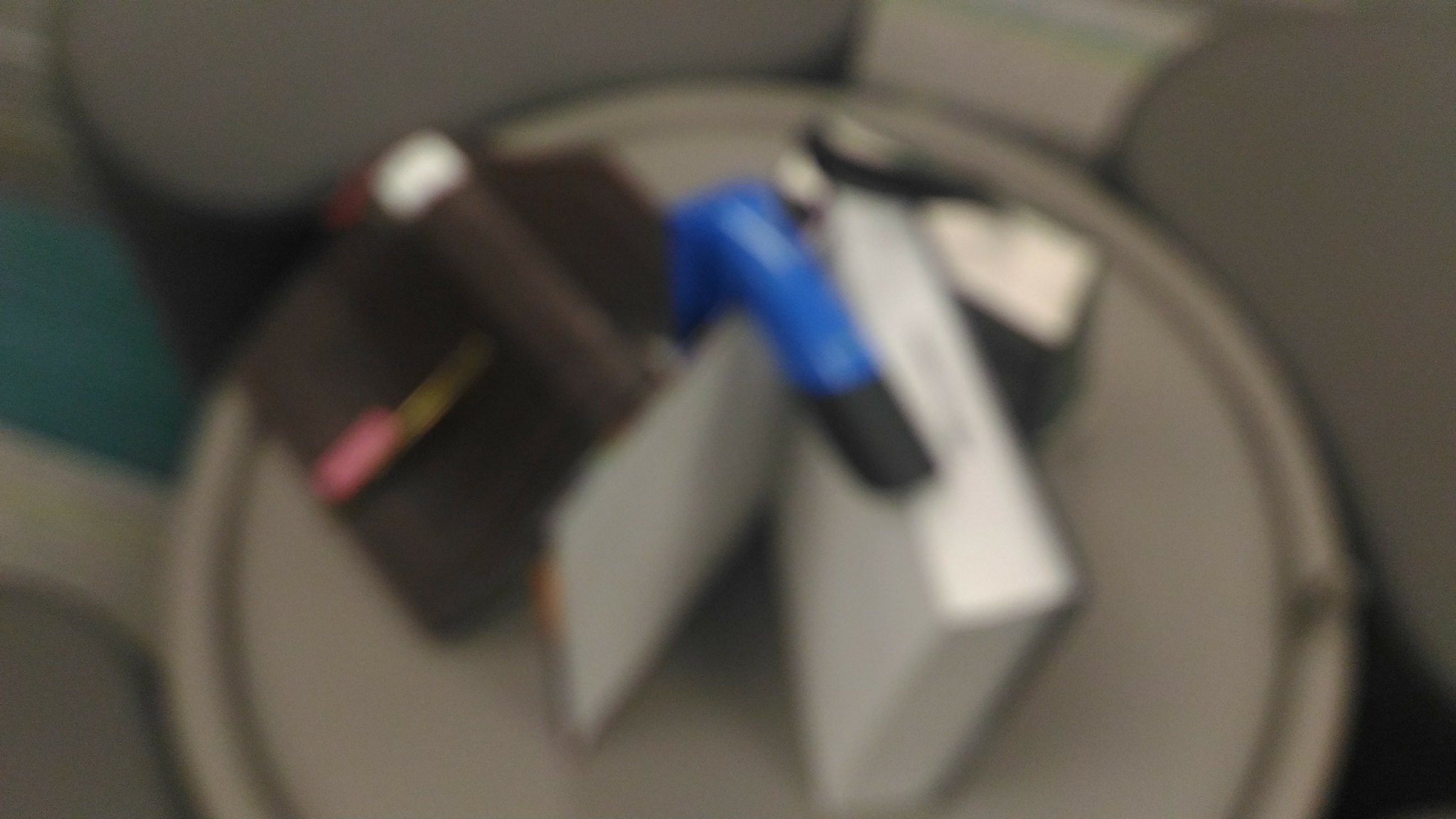The blurred image showcases a cluttered circular coffee table occupying the majority of the frame, positioned up against an L-shaped couch adorned with gray cushions. At the center of the table is a tan circular item with a raised rim, casting a prominent shadow. Several books are scattered across the table: a black book lies face down on the left side, and a white book stands upright in the middle with its cover open, accompanied by a blue and black hand grip strengthening tool draped over it. To the right of this setup, another rectangular, white item, possibly a box or paper, is visible. Behind the central tan object, there's a mix of items, including a black square with a red line and something green, possibly a cushion. The overall scene is extremely out of focus, rendering most objects indistinct and challenging to identify with certainty.